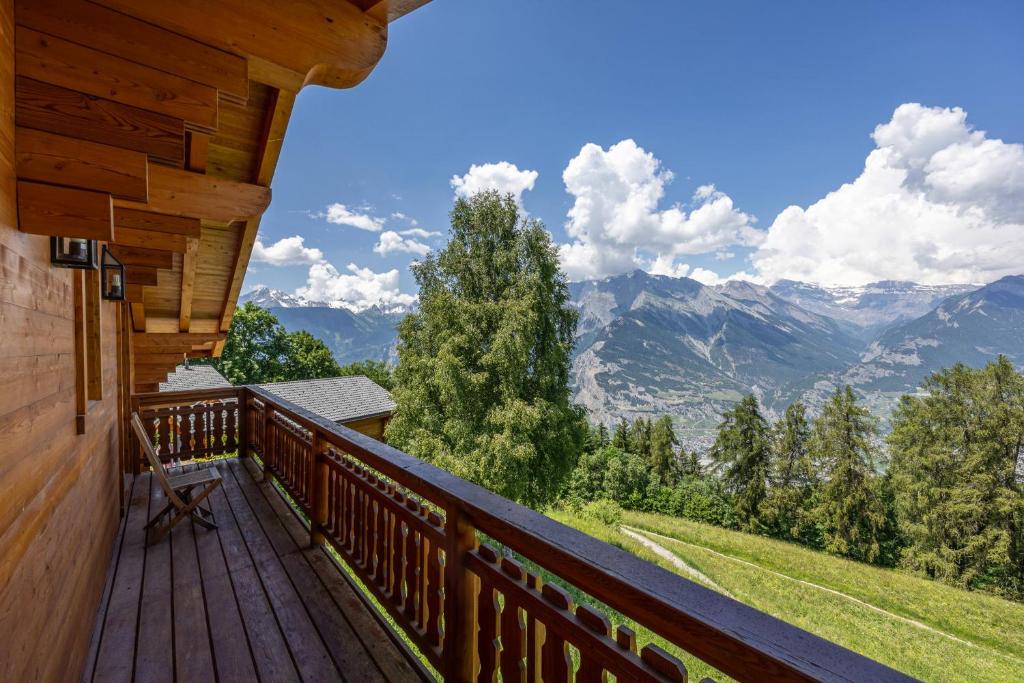This detailed photo captures the serene beauty of a dark wooden cabin from its deck, which overlooks lush green grass and a dense tree line. Prominently visible are two black light fixtures on the left-hand side, and a single chair sitting on the wooden balcony. The sky is a vivid blue, dotted with clouds, as it stretches over the breathtaking mountain range in the background. Beyond the immediate tree line, there is another house partially visible behind the cabin. The photo highlights a beautiful evergreen tree in the foreground and captures the contrasting colors of green and gray in the distant mountains, enveloped by a tranquil, natural setting.